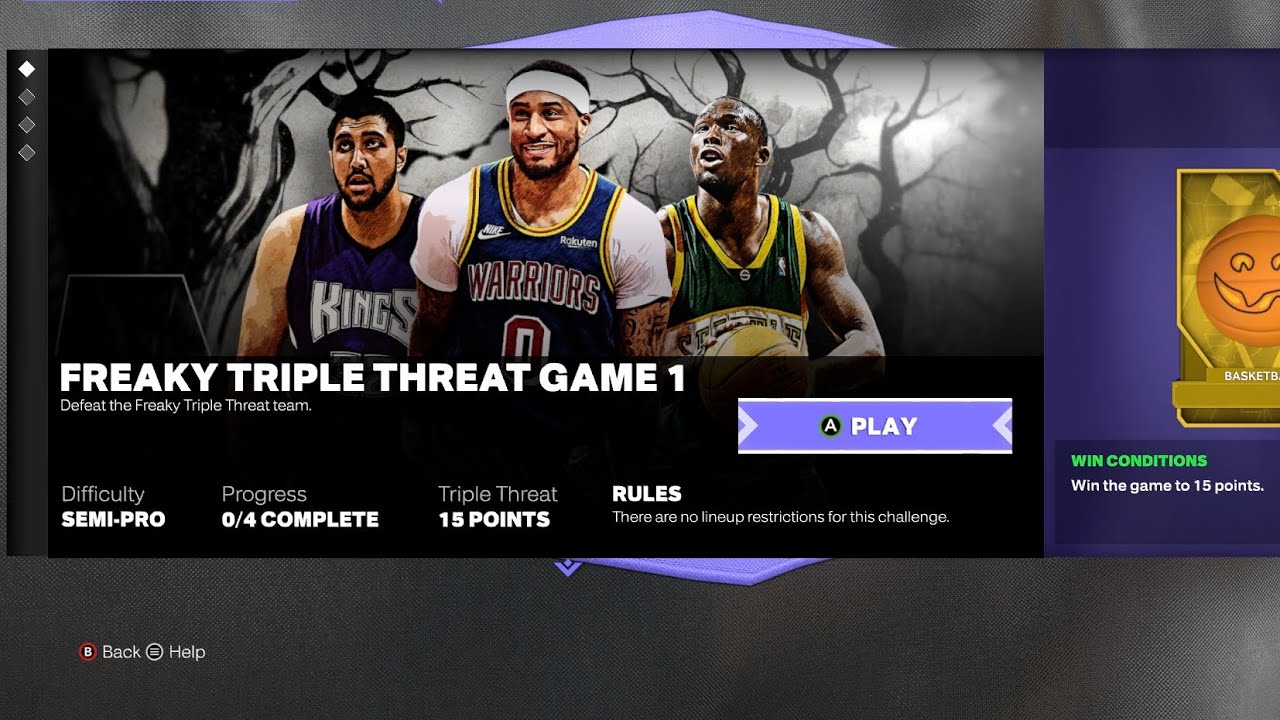Screenshot of a Spooky Basketball Game

This screenshot captures an intense moment in a basketball video game featuring a unique Halloween-themed challenge. The background is a haunting, fog-filled forest, adding an eerie atmosphere to the scene. In the foreground, three players are poised for action, each wearing distinct jerseys: the first player dons a Sacramento Kings jersey, the second sports a Golden State Warriors jersey, and the third player wears a vibrant green jersey.

The challenge is called "Freaky Triple Threat Game 1," where players must defeat the "Freaky Triple Threat Team." The difficulty level is set to semi-pro, with a progress marker currently at 0% complete. The objective is clear: win the game by reaching 15 points. According to the challenge rules, there are no lineup restrictions, encouraging a strategic approach to victory.

The user interface features purple banners above and below the game details, enhancing the spooky theme. On the right side, a basketball with a carved Halloween face is highlighted within a purple outline, adding to the festive vibe. Navigation options include a "Back" button and a "Request Help" feature.

One of the basketball players is captured smiling, seemingly undeterred by the creepy surroundings, ready to take on the challenge.